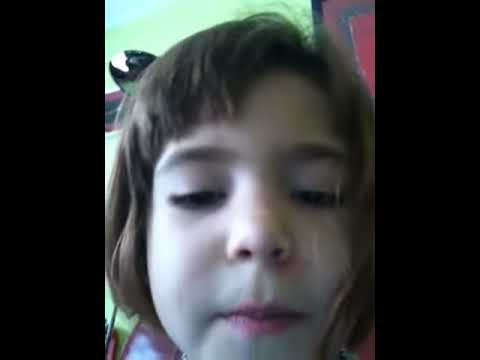This blurred photograph features a close-up of a young girl with fair skin and chubby cheeks, gazing downward, capturing a serene moment. Her medium-brown hair is styled with bangs that are slightly parted, framing her face and running down to shoulder length. She has dark eyes, dark eyebrows, and possibly pink lips, which could be naturally colored or stained from a beverage. The image includes visual elements such as a thick black border on both the left and right sides, giving it a framed effect without borders on the top and bottom. In the background, a green wall is visible, along with a red door in the upper right-hand corner. Lighting from the left side highlights her face, creating subtle shadows on the right, adding depth to the composition. A possible round mirror on the green wall adds an additional point of interest in the scene.